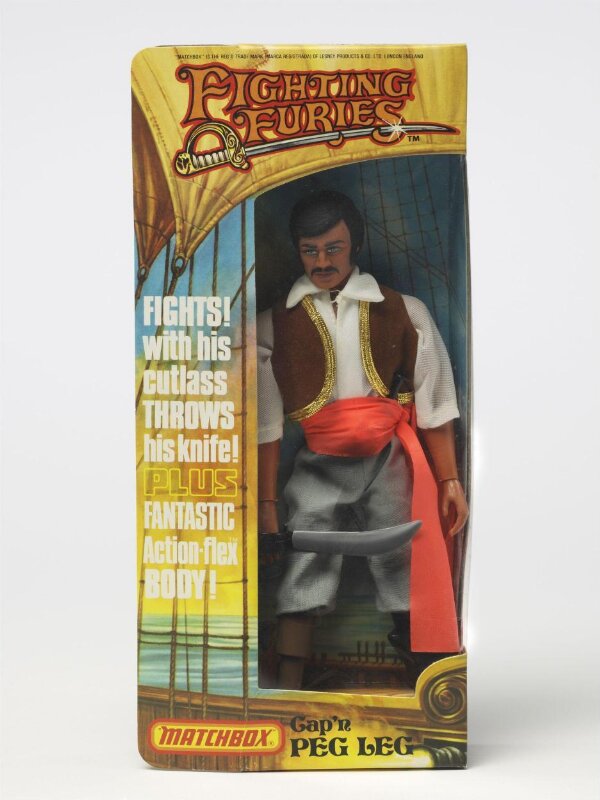The image is a vertically-aligned rectangular picture of an action figure in its original packaging, designed to resemble a pirate. The figure is part of the "Fighting Furies" series, with the title in gold letters outlined in red at the top, accompanied by an image of a sword pointing right. The background features a pirate ship setting in light gray tones.

The action figure itself is visible through a clear plastic window on the right side of the box. He is a dark-skinned man with short black hair, a mustache, and blue eyes. He is dressed in typical pirate attire: a long-sleeve white button-down shirt beneath a brown vest with gold trim, a red or orange sash tied around his waist, gray pants, and tall black boots. He holds a sword or cutlass in his right hand.

Text on the packaging includes “FIGHTS WITH HIS CUTLASS, THROWS HIS KNIFE!” in white letters on the left, with an exclamation mark, and further down, “PLUS FANTASTIC ACTION FLEX BODY” also in white. At the lower left corner, the word "MATCHBOX" is displayed in bold, and to the right, in black lettering, it says "CAPTAIN PEG LEG."

The overall presentation gives a detailed and dramatic impression of an old Matchbox figurine, emphasizing its action features and pirate theme.